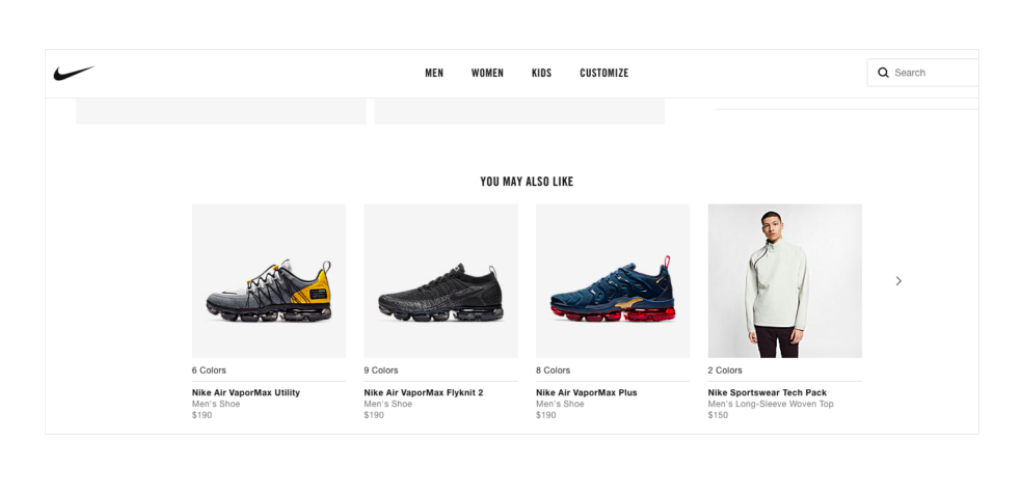At the top left corner is the iconic black Nike swoosh logo. Moving to the right, at the center top, are various navigation subcategories labeled "Men," "Women," "Kids," and "Customize." On the far right, there is a magnifying glass symbol inside the search bar.

Beneath this, in bold black text, it says "You May Also Like." Below this text are four squares arranged horizontally, each showcasing a different Nike product. 

- The first square displays an image of a tennis shoe, which appears to be from the Air Max line. The shoe is gray and yellow with a black outsole and is identified as the Nike Air VaporMax Utility. The shoelaces are black and have a snug fit.

- The second square features a black Nike shoe known as the Nike Air Vaporizer Fly Knit 2.

- The third square highlights a shoe predominantly in navy blue, with a red outsole. This is identified as the Nike Air VaporMax Plus.

- The final square shows an image of a young man, seemingly in his early 20s, with short black hair. He is wearing a long-sleeved white shirt paired with black pants. Underneath this image, it indicates that the outfit is available in "Two Colors" and is part of the "Nike Sportswear Tech Pack," priced at $150.